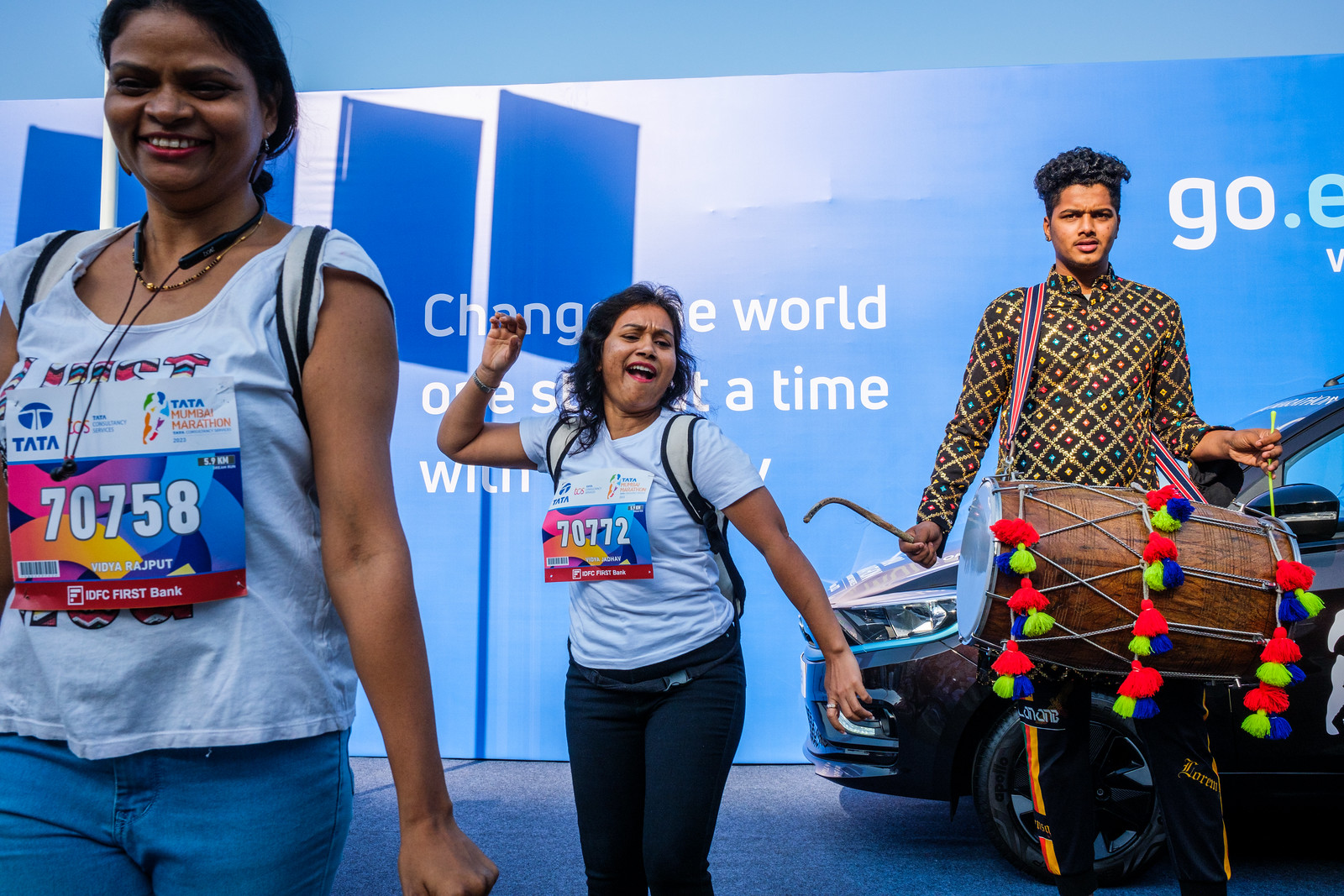The image captures a vibrant scene featuring three Indian individuals set against a backdrop awash in blue hues. A large light blue banner dominates the background, emblazoned with the motivational phrase, "Change the world one step at a time." Positioned in front of this banner are two women and a man.

To the left, a woman with black hair walks forward, donning a light blue tank top and blue jeans. She wears headphones around her neck and has a racing sign taped to her shirt, displaying the number 70758, marked for the Tata Mumbai Marathon with sponsor logos, including Tata.

In the center, another woman in a matching light blue tank top and blue jeans appears to be mid-dance. With her longer black hair cascading down, she raises one arm in the air, her mouth open as if singing or cheering. Her race number, 70772, is similarly taped to her chest.

On the right, a taller man sporting a gold and brown checkered shirt, adorned with colorful accents, plays a barrel drum adorned with red, green, and blue pom-poms. His energetic demeanor complements the lively atmosphere of the scene. 

Together, these elements create a dynamic and spirited depiction of cultural celebration and collective effort.